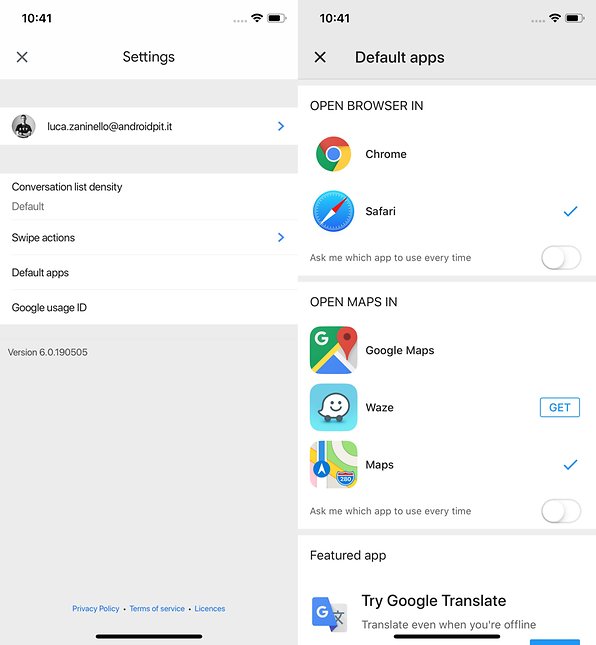This split-screen image shows two illustrations of a mobile phone interface, highlighting various settings and configurations. The top bar of both images displays the time as 10:41, with Wi-Fi and battery icons shown on the right side. On the left, the word "Settings" is visible, accompanied by an 'X' icon. 

The main focus features a profile section, showing the name "Luca de Zaninello" with an associated email, "androidpit.it," and a small, circular, black-and-white profile picture of a man. Below the profile, there's a list of customizable options including "Conversion List Density," "Swipe Actions," "Default Apps," and "Google Usage ID."

On the right side, an expanded view of the "Default Apps" settings is displayed. It includes options for opening browsers and maps. For browsers, there is a choice between "Chrome" and "Safari," with Safari selected and a statement indicating the user will not be prompted to select an app every time—this option is turned off. Similarly, map applications can be chosen between "Google Maps," "Waze," and "Maps," with the Maps app selected, and an option to ask each time being checked.

At the bottom of the screen, there is a recommendation to try the "Google Translate" app, along with its icon and the feature note, "Translate even when you're offline."